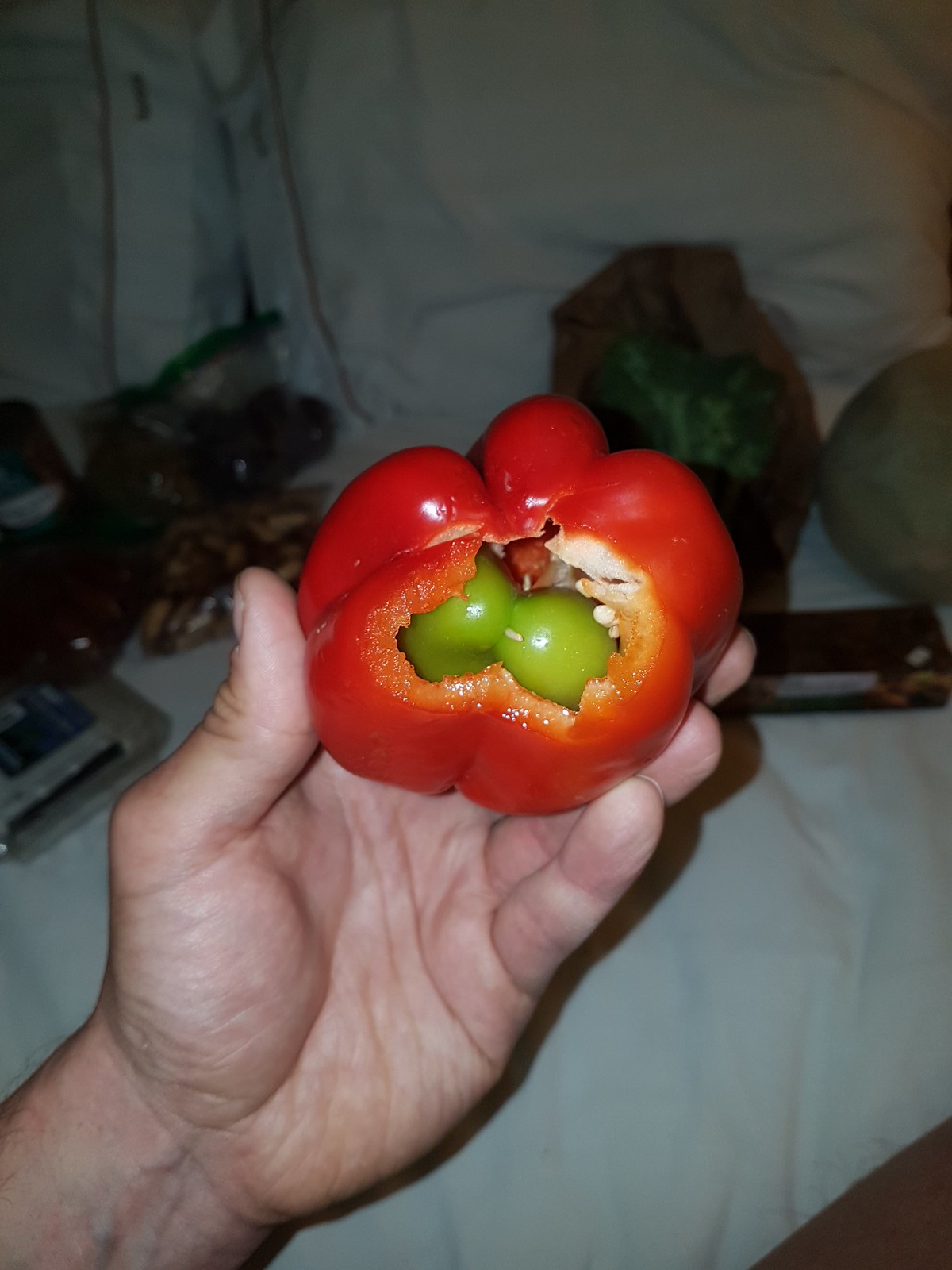A left hand, appearing large and likely male, holds a red bell pepper with a chunk missing from its bottom. This reveals an unusual sight: a smaller, green bell pepper growing inside the red pepper. The textured skin of the peppers contrasts vividly. In the background, a bed with white pillows and sheets is visible, scattered with various vegetables and fruits. To the right, there's a blurry item that might be melon or cabbage. On the left, a paper brown bag rests with a head of green broccoli on top, and beneath it is a burgundy-colored food box. Additional bags filled with fruits clutter the left side. The image focuses sharply on the peculiar pepper phenomenon, while the background remains unfocused, adding to the intrigue of the scene's disorganized appearance.